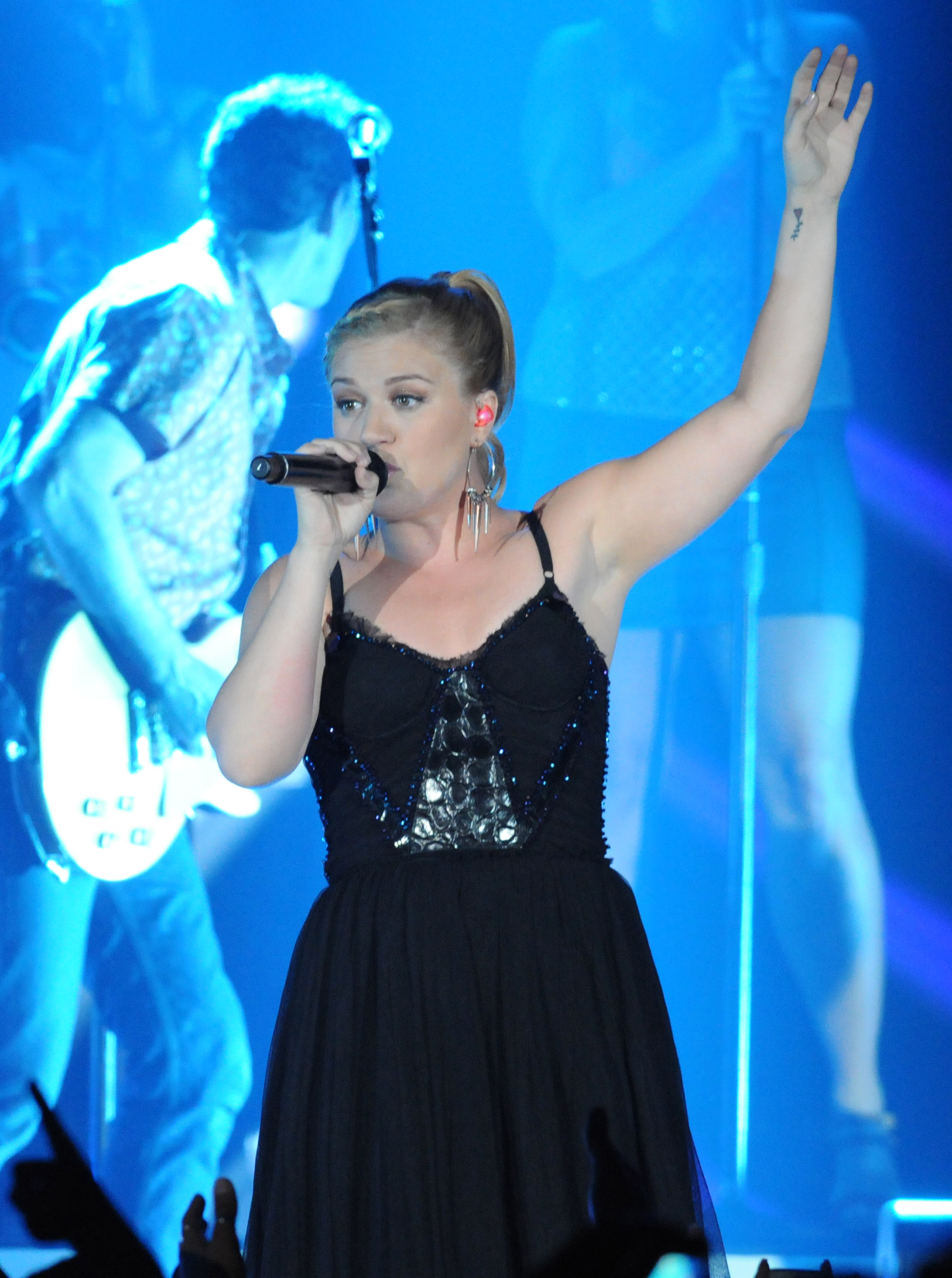In this image, we observe a dynamic concert scene, with a striking blue spotlight creating a vibrant backdrop. Dominating the center stage, a woman in a black dress with glitter and sequins detail on the top, and pleats on the bottom, holds a microphone aloft, standing confidently. She faces forward, but her head is turned slightly to the left. Behind her, a man plays a white electric guitar; he wears jeans and a short-sleeved polo shirt, his short hair visible as he gazes away towards the back and right of the picture. Off to the right in the background, there is another woman, partially obscured, wearing shorts. There's no text present in the image, and the dominant colors include shades of blue, black, white, gray, and tan, suggesting the event likely takes place indoors, amidst a lively musical performance.